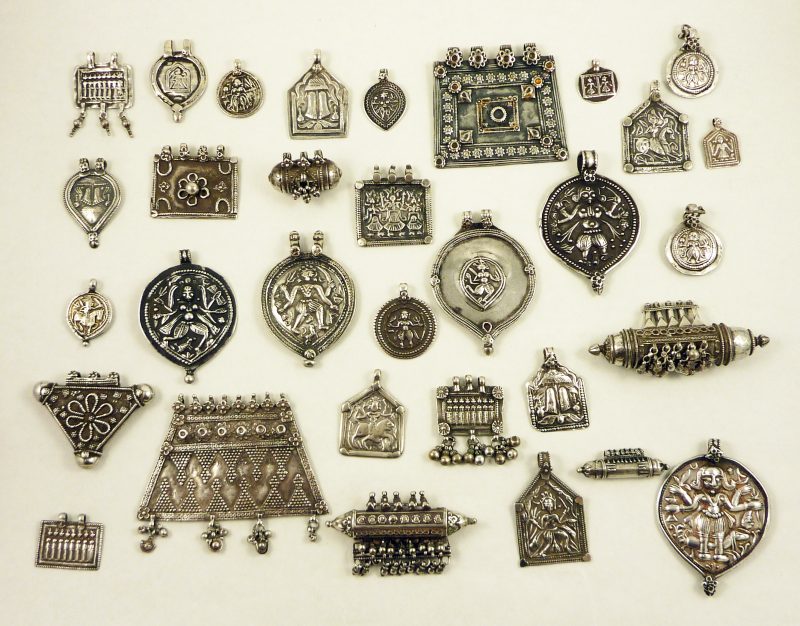The image displays an array of antique silver jewelry meticulously arranged on a beige background. These pieces include pendants and medallions of various shapes such as oval, circular, rectangular, trapezoidal, and teardrop, all featuring intricate designs. The largest piece, positioned second from the left on the bottom row, has a championship-like shape adorned with triangular and circular patterns. Beneath it, four smaller pendants dangle from its base. On the bottom right corner, an oval pendant depicts a heavily embossed humanoid figure with four arms, dressed in a distinct skirt, possibly straw. The artifacts exhibit a mix of silver and bronze hues due to lighting variations, and many pieces feature figures with multiple arms, suggesting an Indian influence. Both large and small, each piece is equipped with hooks for wearing as necklaces, highlighting their potential use as personal adornments.